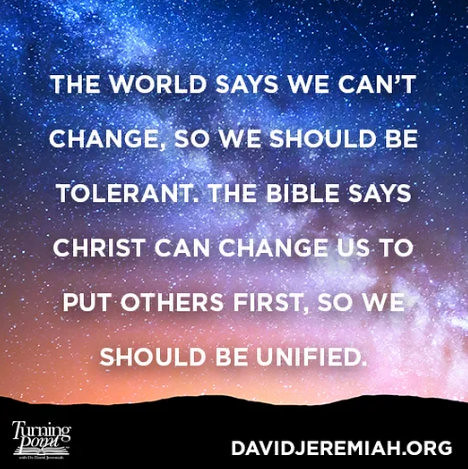The image is a photograph featuring a long-exposure shot of the night sky, dotted with stars and showcasing the Milky Way. As the sky descends towards the horizon, it transitions into hues of orange and pink, eventually meeting a solid black strip of silhouetted mountains at the bottom. Centered against this celestial backdrop is a quote in all-capital, white, sans-serif letters stating: "THE WORLD SAYS WE CAN'T CHANGE, SO WE SHOULD BE TOLERANT. THE BIBLE SAYS CHRIST CAN CHANGE US TO PUT OTHERS FIRST, SO WE SHOULD BE UNIFIED." In the bottom right corner, the website "davidjeremiah.org" is printed, while the lower left corner features the "Turning Point" logo, which includes an image of an open book.